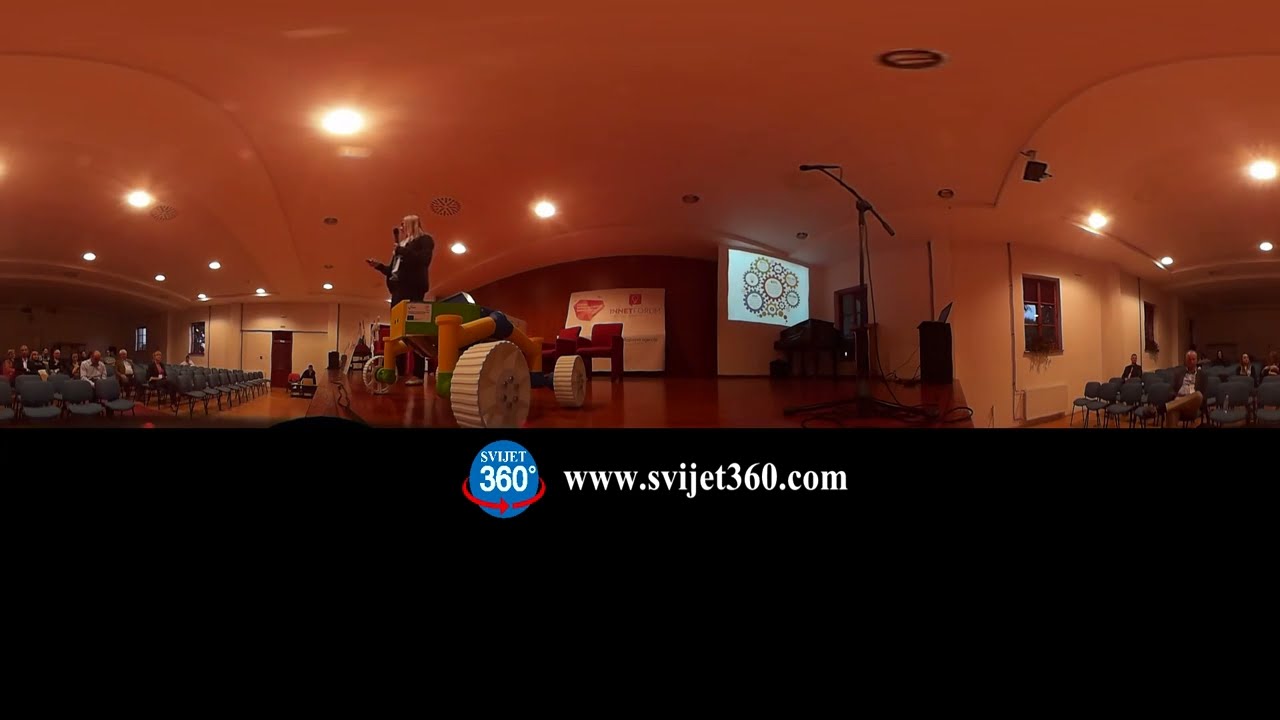The image depicts a scene from a conference or meeting room. At the bottom of the image, there is a black bar featuring a blue circle with white letters spelling "SVIJET" and "360" beneath it. A red arrow encircles the blue circle in a counterclockwise direction, forming the logo. To the right, in white font, the website "www.svijet360.com" is displayed. Above this, the stage area is visible, showing a person in a black coat and black pants holding a microphone and looking down at a tablet. The person appears to be a female speaker. The room is organized with blue chairs arranged in orderly rows, and there are additional chairs and microphones on the stage. A white projector screen is present, lit by the overhead ceiling lights, enhancing the professional setting of the meeting room.